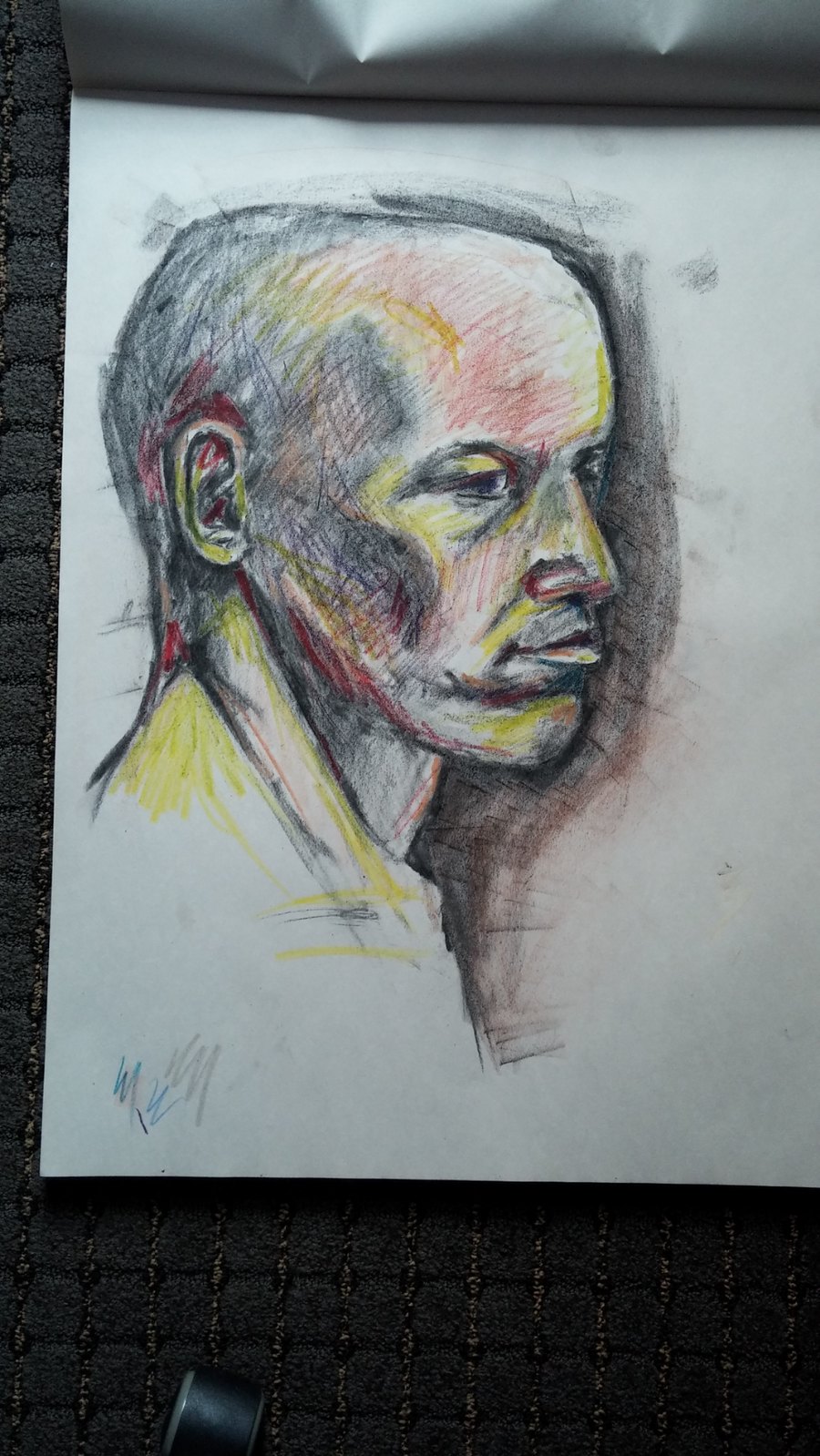A detailed and expressive sketch drawn on a white sheet of sketch paper, which rests on a dark surface, possibly a black paneled desk. The artwork, created using colored pencils and charcoal, portrays the somber profile of a man with a receding hairline, his head turned slightly towards the right. His face, neck, and a portion of his collared shirt are meticulously shaded, with generous use of blacks to intensify the shadows and create a sense of depth. The man's expression is notably grumpy, further emphasized by the dark shading surrounding his face, which augments his look of misery. Bold splashes of color—including bright reds, purples, and yellows—are used to highlight his facial tones, suggesting underlying emotions of pain and depression. The artist's signature, "W.W.," is discreetly placed in the bottom left corner of the paper.